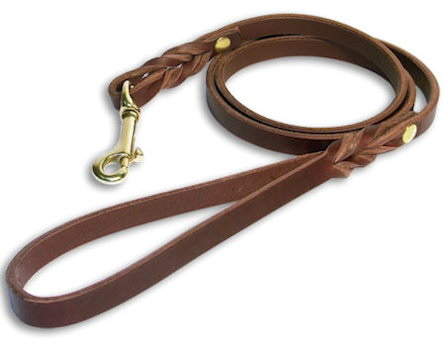This detailed photographic image captures a rich, chocolate brown leather strap, likely intended as a leash or harness, showcased against a pristine white background. The strap, positioned diagonally from the bottom left corner to the top right and coiled into several loops, displays its robust and thick material. The ends of the strap feature intricately braided sections, each secured by brass buttons, suggesting they were hammered into place. At one end, a brass or yellow-colored spring-loaded carabiner, commonly used for keychains, adds a functional touch, emphasizing its potential use for animals such as dogs. The strap’s overall design, with its multiple loops and gold-colored accents, highlights craftsmanship and practicality, all beautifully illuminated by a direct overhead light source, enhancing its fine details and texture.